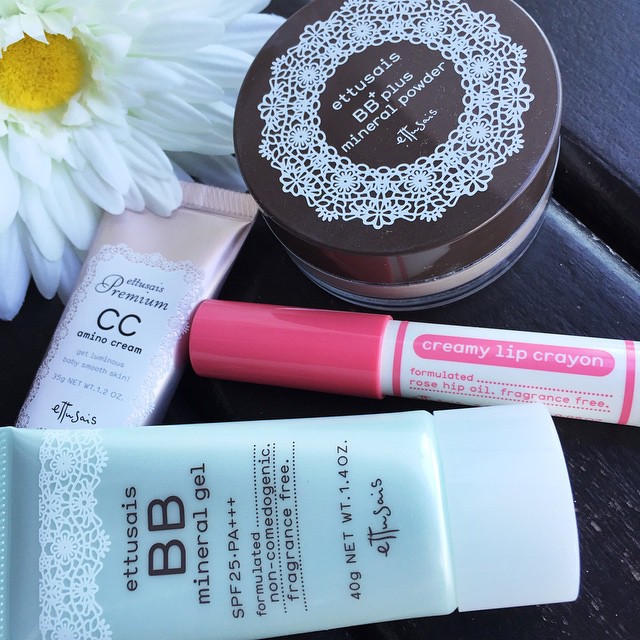The photograph, presented in a square format, showcases an artistic arrangement of cosmetic toiletries on a black table. Dominating the top left corner of the image is a large, partially cropped white daisy with a vibrant yellow center, adding a touch of natural beauty to the scene. In the foreground, a selection of skincare products is meticulously positioned. 

To the left, there is a tube of BB mineral gel featuring a delicate white lace motif near the top; the text "BB Mineral Gel" is displayed in bold black lettering with additional details beneath. Adjacent to this is another tube, pale pink with similar lace detailing and labeled "CC Amino Cream." Both tubes are lying on their sides, emphasizing their design and text.

On the top right, a large container of BB Plus Mineral Powder stands upright, capped with a brown lid. Its clear circular base reveals the powder inside, and the lid has a prominent white lace design with "BB Plus Mineral Powder" inscribed in elegant white letters. Just below this container, a creamy lip crayon in a lighter pink shade completes the arrangement, its packaging adorned with intricate text stating "Creamy Lip Crayon."

The overall composition, heightened by the natural element of the daisy and the intentional grouping of the products, suggests a carefully curated collection likely intended for a product package or artistic presentation.